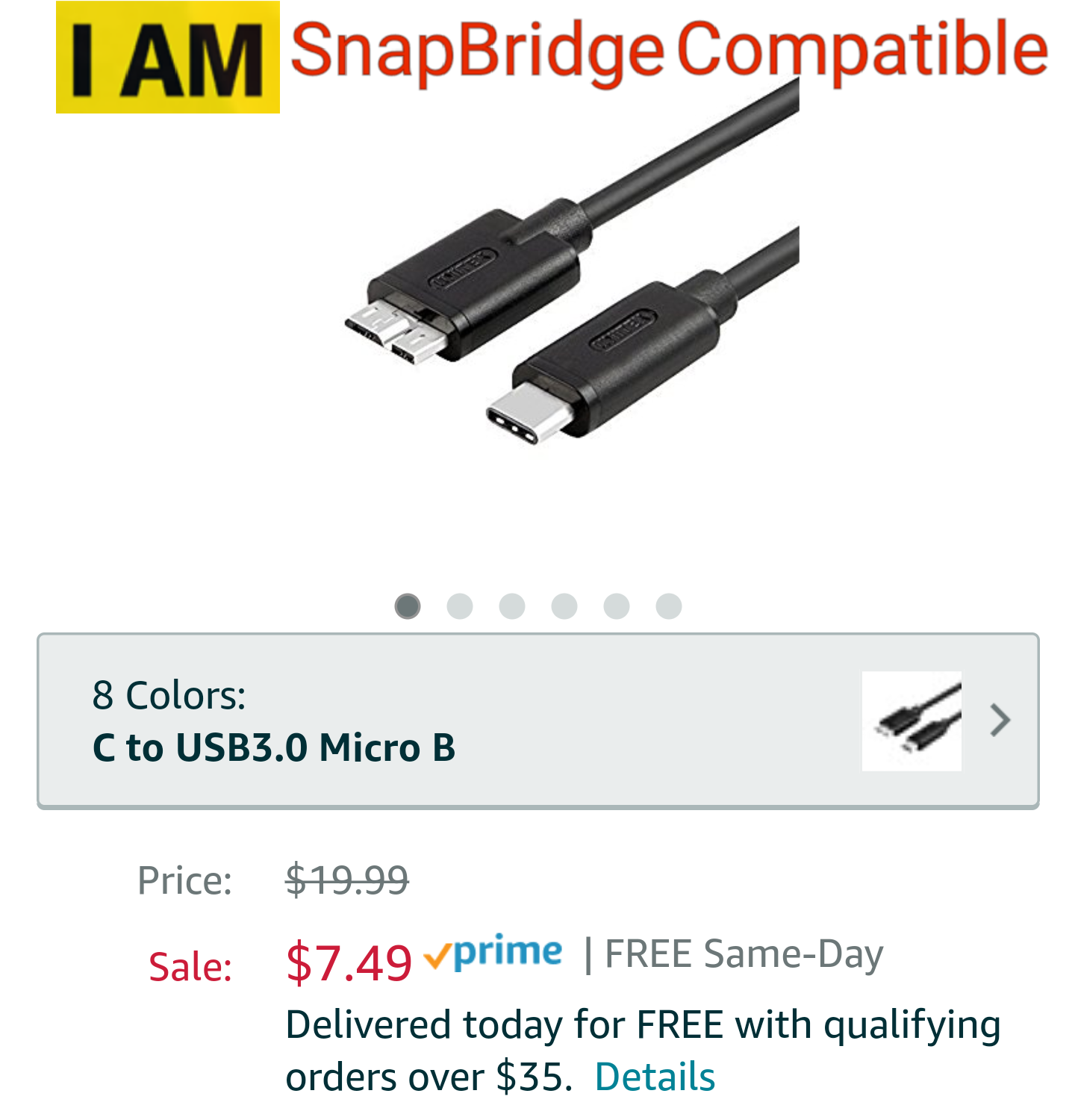This image is a cropped and edited screenshot from the Amazon.com mobile app. The top of the image features a yellow box with the words "I am" in black text, positioned to the left. To the right, "Snapbridge compatible" is displayed in red text. The usual header for product listings is cut off at the top.

In the center of the screenshot, there is a large thumbnail image showcasing two ends of a cable. Directly below the thumbnail, there are six grey dots aligned horizontally, with the first dot shaded in a darker grey to indicate that the current thumbnail is the first photo.

Beneath this row of dots, a large grey rectangle features the text "Eight colors," and below that, it specifies "C to USB 3.0 micro B" in smaller text. To the right, there is an arrow pointing left, indicating an option to switch colors. A smaller thumbnail of the main image is adjacent to this arrow.

Towards the bottom of the screenshot, the original price of the product, "$19.99," is displayed in grey and crossed out. Below this, the word "Sale" appears in red text, with the discounted price of "$7.49" shown next to it in red. To the right of the discounted price, the Prime logo is visible, accompanied by the text "Free Same-Day" in large grey letters. Directly below, it states "Delivered today for free with qualifying orders over $35.00," followed by the word "Details" in blue hyperlink font.